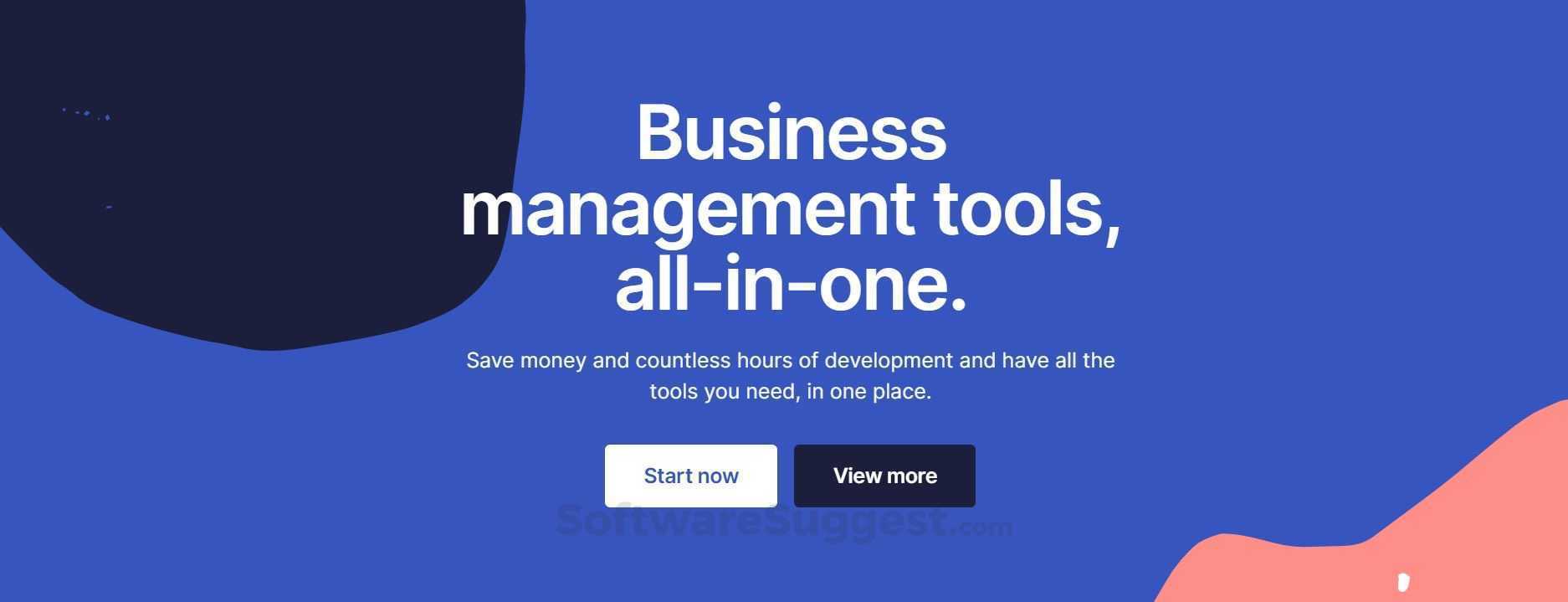Here is a cleaned-up and detailed caption for the image:

"A screenshot of an advertisement from SoftwareSuggest.com featuring a gradient blue background that transitions from dark to light shades. In the upper left corner, a dark navy blue bubble contains white text that reads, 'Business Manager Tools - All-in-One.' Below, it states, 'Save money and countless hours of development with all the tools you need in one place.' There are two buttons at the bottom of the bubble: a white button labeled 'Start Now' and a black button labeled 'Learn More.' A watermark from SoftwareSuggest.com is visible. In the bottom right corner of the image, there is a peach-colored blob with a small white dot in its center, adding a touch of contrast to the overall design."